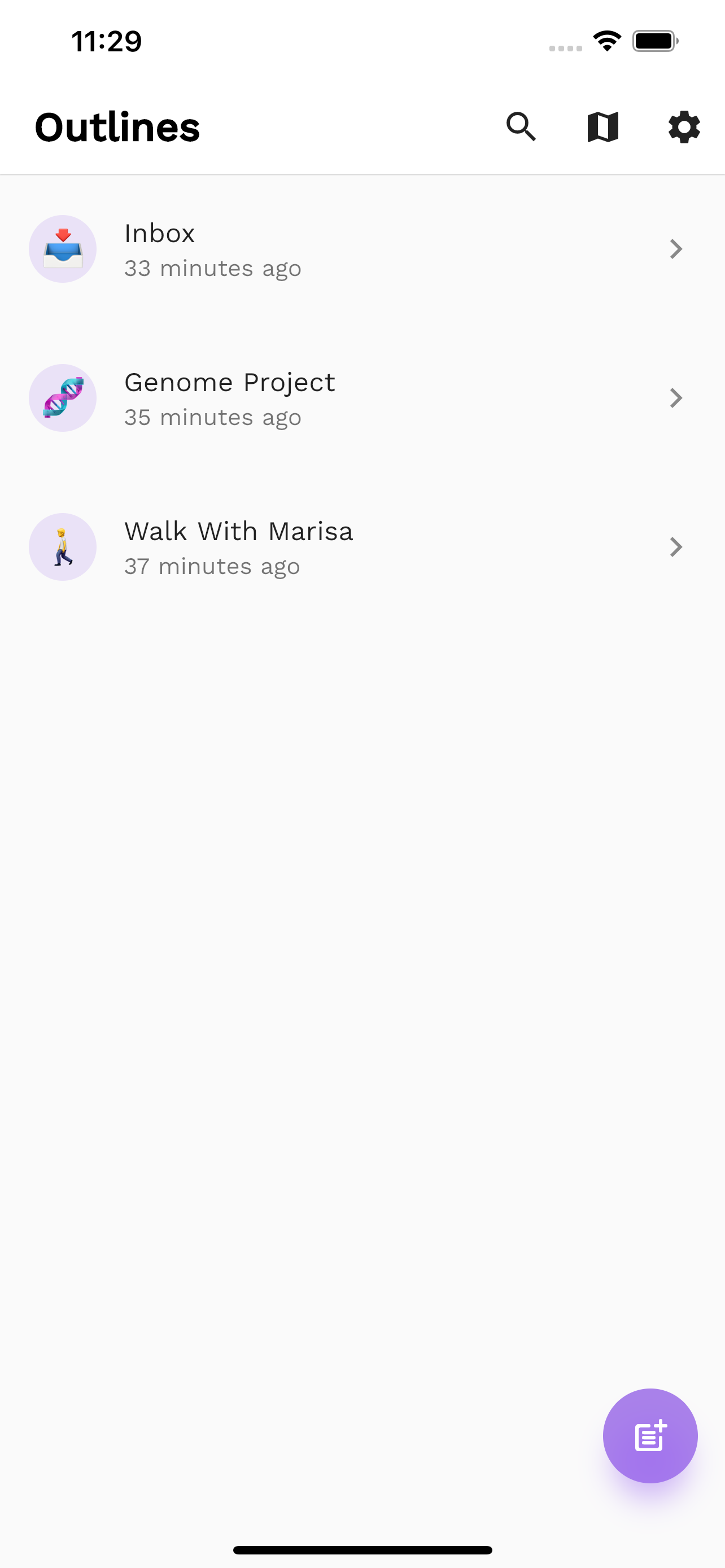This image is a screenshot taken from a phone or tablet device displaying an application titled "Outlines." At the top of the screen, the time is indicated as 11:29. Additionally, on the top left, there are four dots, a Wi-Fi signal icon, and a fully charged battery icon, signifying the device's status.

The main heading "Outlines" is prominently displayed in bold black text. Below this heading, there is a divider that separates it from three sections listed underneath.

1. The first section is labeled "Inbox," with a timestamp indicating "33 minutes ago" and an icon to the right suggesting more details can be accessed.

2. The second section is titled "G.E. and O.M.E. Project," marked as "35 minutes ago," again with a clickable icon on the right.

3. The third section reads "Walk with Marissa," noted as "37 minutes ago," with an option to view more details to the right.

At the very bottom of the page, there is an icon that looks like a box containing three horizontal bars, and within this box, there is a plus sign, implying the functionality to add new items or sections.